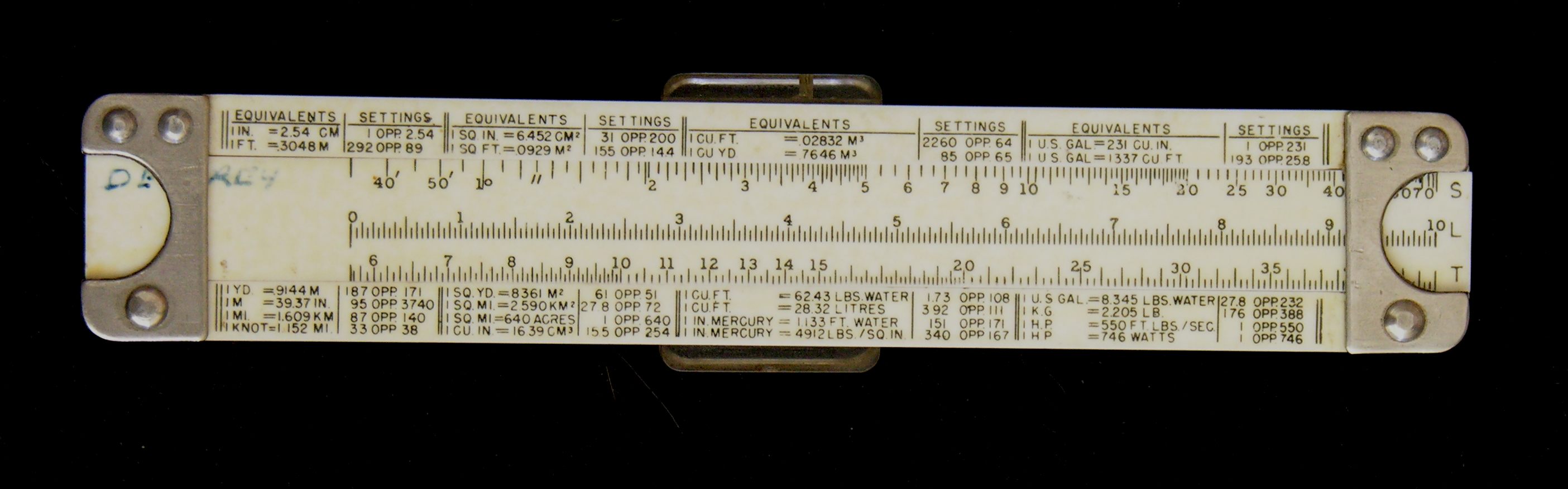This image depicts an antique, rectangular measuring tool that resembles a ruler. The background is a solid black, accentuating the details of the instrument. The ruler itself is primarily made of white plastic, featuring black writing and numbers. Metal end caps are situated on both the right and left ends of the tool, providing durability and an old-fashioned aesthetic. 

The top section of the ruler showcases a series of text, starting with the word "equivalents" prominently in the left middle area and repeating "settings, equivalents, settings" horizontally. Below this section, there are various numerical markings akin to traditional ruler measurements, spanning from 0 to 10 inches. Additionally, the ruler includes a conversion scale, with various units such as "YD" (yards), "M" (meters), and "MM" (millimeters) marked on it. This conversion scale is indicative of its utility for various measurement conversions, including inches to centimeters (1 inch equals 2.54 centimeters) and feet to meters (1 foot equals 3,400 centimeters), among others.

Notably, there is blue ink writing near the far left end of the ruler, although partially obscured, with letters like "DRC4" faintly visible at both the top and bottom. The central lower portion of the ruler appears to have additional metal parts, possibly clips or buckles, adding to its multifunctional design. This measuring tool is not just a simple ruler but a comprehensive utility tool with multiple measurement conversions and formulas, indicating its extensive usage in various settings.